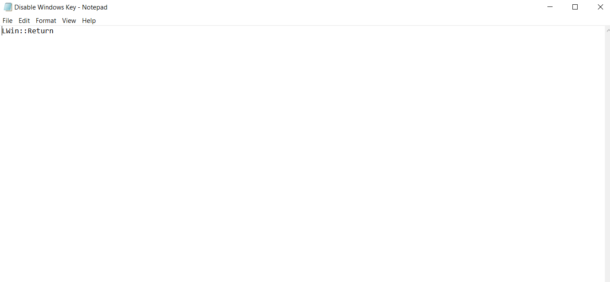This image depicts a screenshot of a text editing application on a computer. The interface is predominantly clean with a prominent white header at the top spanning the entire width. On the far left of the header, a blue notepad icon is displayed. Adjacent to the icon is the text "Disable Windows Key - Notepad" in gray. Further left, there are five menu options in medium gray text: "File," "Edit," "Format," "View," and "Help." A substantial portion of the header consists of negative white space. On the top right, there are three functional icons: a minus icon for minimizing, a square outline icon for maximizing, and an 'X' icon for closing the application.

A very thin light gray line divides the header from the main body of the document. The body features a pristine white background. Positioned at the top left of the body section is the text: "LWIN:: return" in dark gray, with "LWIN" and "R" capitalized. The placement of a vertical gray line signifies the cursor's position on the left side. On the far right side of the body, a light gray scroll bar is visible, featuring a medium gray upward-pointing arrow at its top.